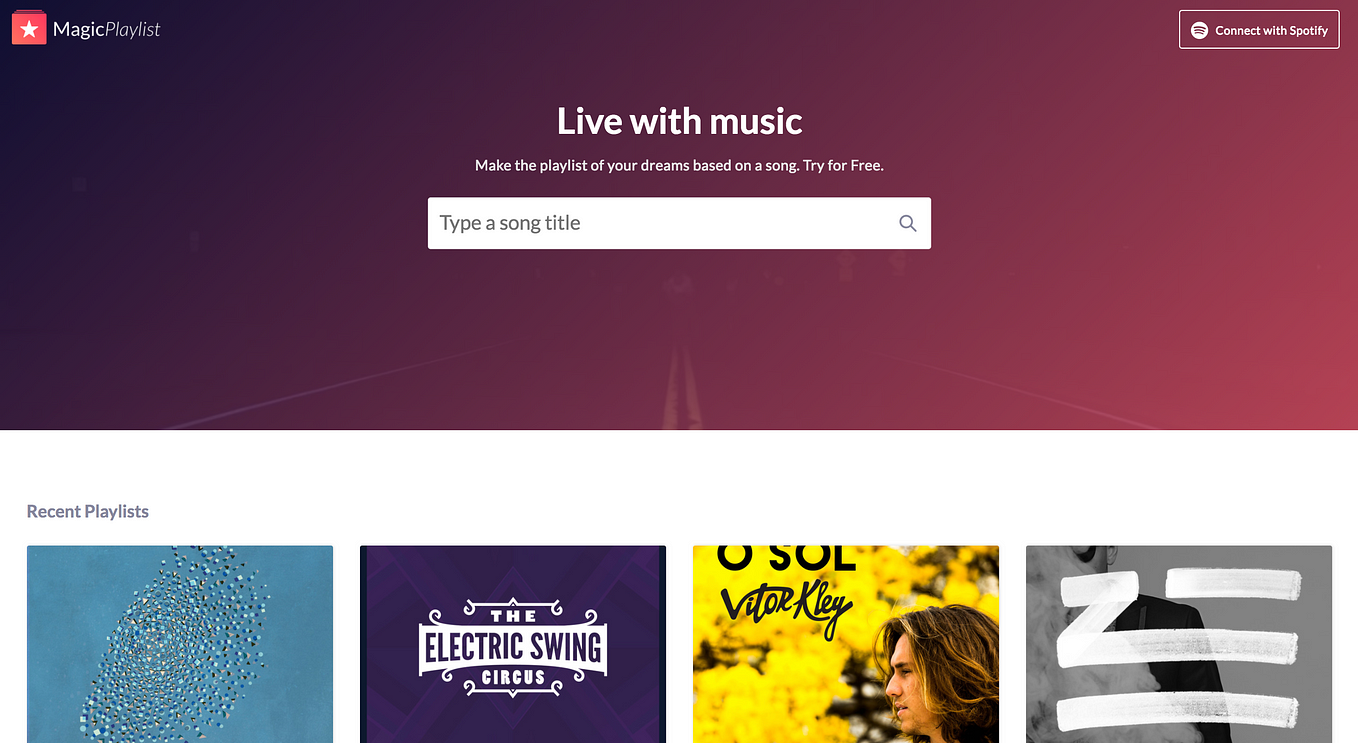This image appears to be a screen capture from a music-related app or website interface. At the top of the image is a large rectangular section split between a deep purple color and a moth-like graphic. In the top-left corner of this rectangle, there is a red square featuring a white star, labeled "Magic Playlist." On the opposite corner, there is a white box with the text "Connect with Spotify." 

Central to this purple and moth-like background is a prominent tagline that reads, "Live with Music. Make the Playlist of Your Dreams Based on a Song. Try for Free." Below this, there is a white input box with the placeholder text "Type a song title," accompanied by a gray magnifying glass icon indicating a search function.

Directly beneath this section, the heading "Recent Playlist" is displayed in gray. Below this heading, there are four square images arranged in a grid pattern. 

1. The first image is in a darker shade of baby blue, featuring multicolored pebbly elements in tan, black, and blue.
2. The second image features a purple background with the text "The Electric Swing Circus" in white and purple font.
3. The third image shows yellow leaves and a person with light skin and brown hair, alongside the text "Osawa Victor Clay" in black font.
4. The fourth image contains a gray square with white graffiti-style artwork resembling an abstract person in the backdrop.

Overall, the image visually conveys a vibrant and engaging user interface dedicated to music playlist creation and discovery, with a blend of colorful and artistic elements.